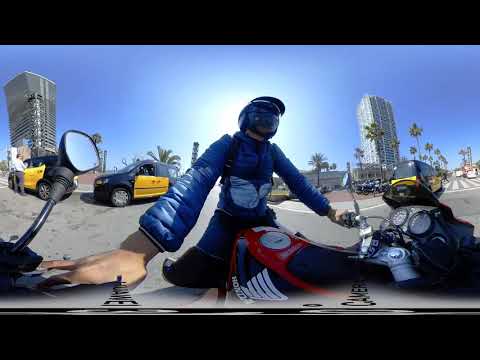The image showcases a person in the center, fully visible and wearing a blue mask, a black cap, and a blue puffer jacket. They have a white bag strapped to their chest and are holding onto two motorcycles. The left motorcycle is only partly visible, with its front mirror standing out, whereas the right motorcycle is red and black. The individual’s left hand is holding the throttle of the right motorcycle. Distortion affects the person’s right arm, hand, lower body, and the back of the motorcycle on the right.

Surrounding this central figure is a street scene. Behind the person is a road with three vehicles, including a notable yellow and black DHL van to the left center. Additionally, a yellow bus can be seen to the right, along with other parked cars. The background reveals a blue sky with white sunlight illuminating the scene, two tall buildings—one on each side of the image—and some palm trees near a crosswalk. The image is framed with thick black borders at the top and bottom, embellished along the bottom with three emblems: a black one on the left, a white one in the middle, and a black one on the right.